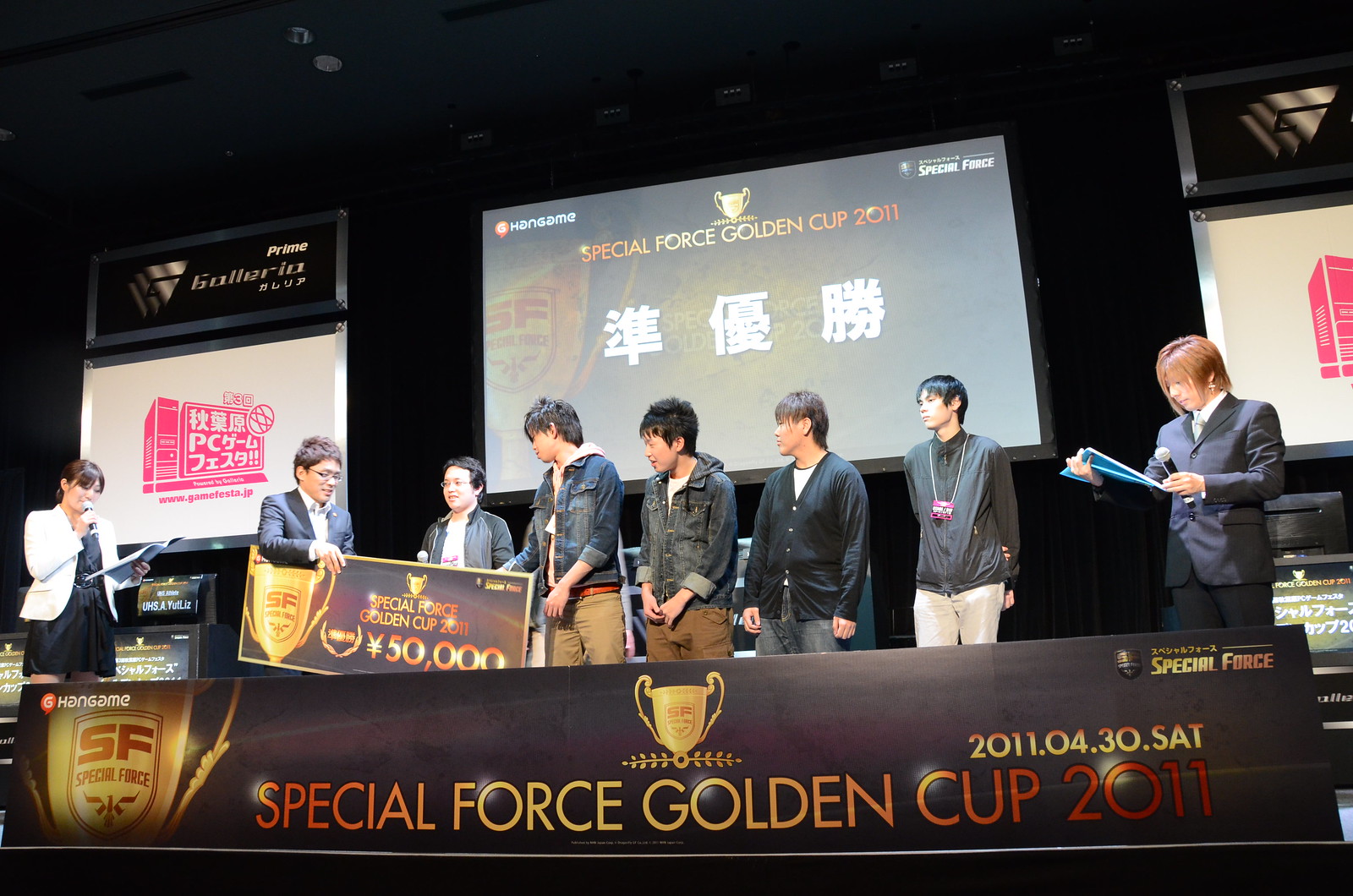The photograph depicts an indoor awards ceremony, likely at an eSports event called the Special Force Golden Cup 2011. The stage features a group of young men, presumably in their late teens, all of whom appear to be Asian and dressed casually in streetwear, including jean jackets. They are flanked by two individuals in formal attire; on the far left is an Asian woman wearing a black dress with a white jacket, holding a microphone and reading from an open booklet. To the far right stands another man in a suit, also holding a microphone and a booklet. A central figure in a suit is handing the young men a large black check adorned with a golden trophy design, signifying their award of 50,000 yen. The backdrop includes a banner and a projector display, both prominently featuring the text and logo of the Special Force Golden Cup 2011.